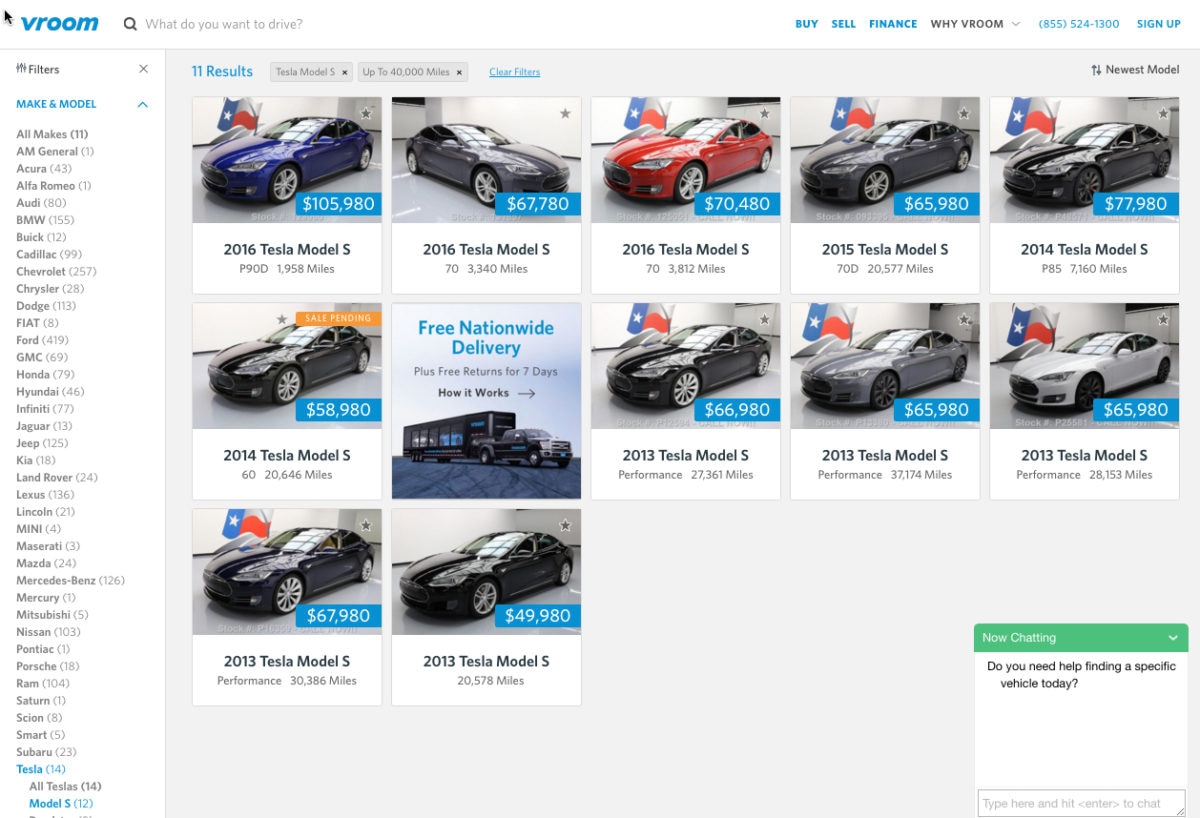The image is a screenshot from a car sales website branded "Vroom," prominently displayed in blue on the left side. At the top of the page is a search bar with the prompt, "What do you want to drive?" On the right side, in blue text, it lists options for "Buy, Sell, Finance," and a customer service number "(855) 524-1300," along with a "Sign Up" button. The section labeled "Why Vroom?" is in black and includes a dropdown arrow.

The main content shows a filtered search result for Tesla Model S cars with up to 40,000 miles. There are 12 squares with car listings, although only 11 are images of cars. Here's a detailed breakdown:

1. A blue 2016 Tesla Model S P90D with 1,858 miles, priced at $105,980.
2. A grey 2016 Tesla Model S 70 with 3,340 miles, priced at $67,780.
3. A red 2016 Tesla Model S 70 with 3,812 miles, priced at $70,480.
4. Another grey 2015 Tesla Model S 70D with 20,577 miles, priced at $65,980.
5. A black 2014 Tesla Model S P85 with 7,160 miles, priced at $77,980.
6. Another black 2014 Tesla Model S displaying "Sale Pending" in orange. It has 20,646 miles and is listed for $58,980.
7. An informational square stating "Free nationwide delivery plus free returns for 7 days" with an illustration of a truck pulling a trailer, labeled "How it works".
8. A black 2013 Tesla Model S Performance with 27,361 miles, priced at $66,980.
9. A light-grey or possibly dusty blue 2013 Tesla Model S Performance with 37,174 miles, priced at $65,980.
10. A white 2013 Tesla Model S Performance with 28,153 miles, priced at $65,980.
11. A black 2013 Tesla Model S Performance with 30,386 miles, priced at $67,980.
12. Another black 2013 Tesla Model S with 20,578 miles, priced at $49,980.

Additionally, there is a chat box on the bottom right with a green dropdown reading "Now Chatting." The white text box within the chat asks, "Do you need help finding a specific vehicle today?" allowing users to chat with a representative.

The website offers a wide selection of vehicles beyond Teslas, including brands such as Acura, BMW, Mercury, Scion, Nissan, and Mazda, suggesting a diverse inventory for potential buyers.